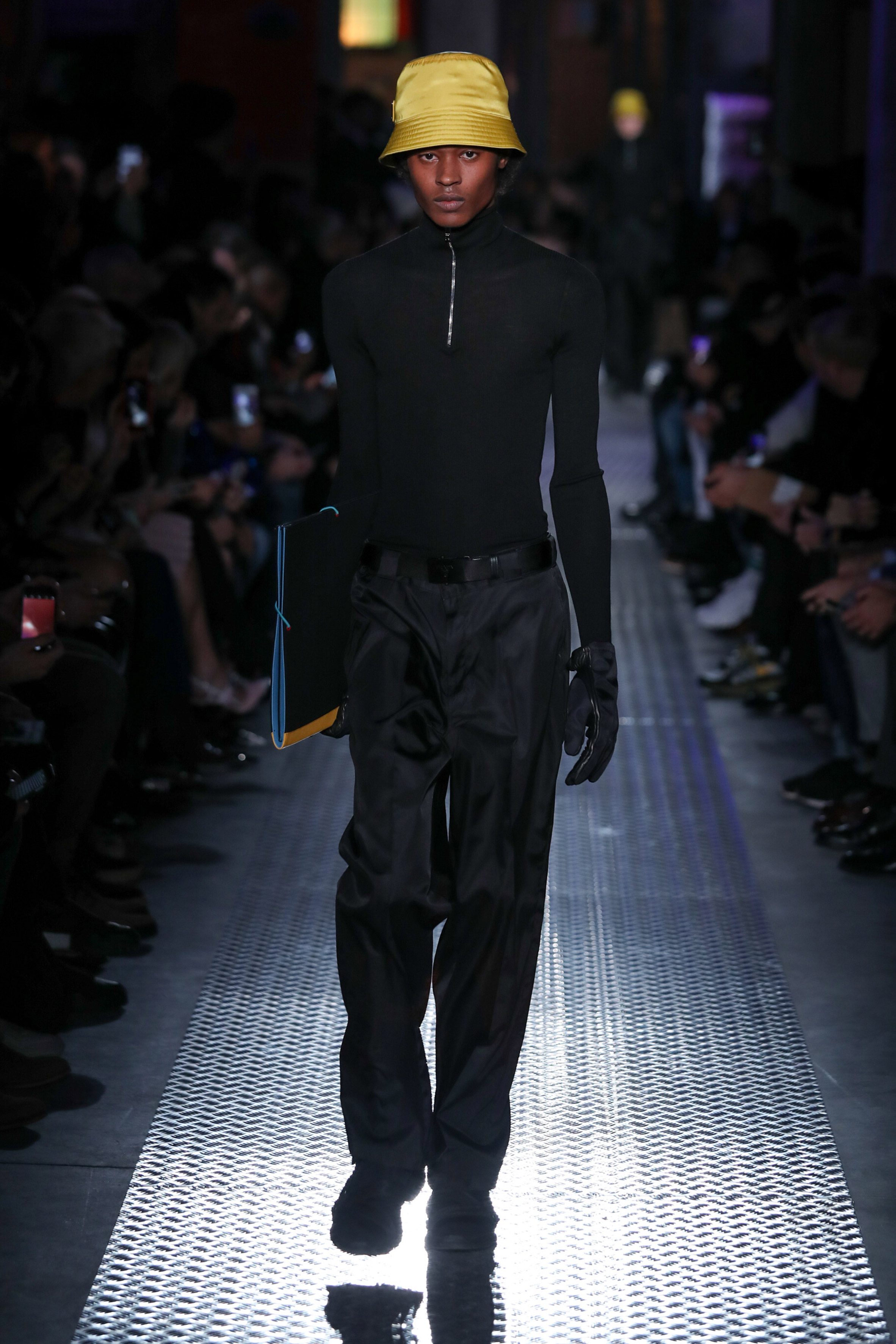This photograph captures a tall, slender male model with dark brown skin walking down a metallic, industrial-looking runway at an indoor fashion show. The model is moving towards the viewer, and flanking the runway, we can see the blurred feet and hands of audience members seated in dim lighting, possibly capturing the moment with their phones. The model exudes a serious demeanor, donning a distinctive yellow bucket hat with horizontal ripples, a fitted black high-neck quarter-zip sweater, and loose, shiny black pants secured with a black belt. He completes the ensemble with black boots and holds black gloves in one hand, while carrying a black portfolio with brown binding and blue edges in the other, emphasizing the overall monochromatic theme punctuated by the striking yellow hat.